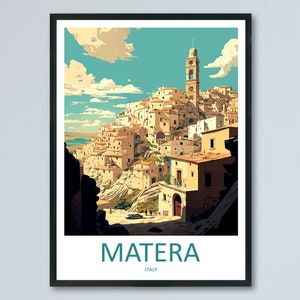On a light gray wall hangs a beautifully framed painting in a sleek black rectangular frame. The painting features a picturesque coastal Mediterranean-style city, identified as Matera, Italy. Encased within a white border, the peaceful scene depicts a village of tan, stucco-like buildings built into a hillside. Above the town, a bright blue sky is dotted with a few fluffy white clouds. The buildings are distinctive with their light tan stone facades, including a prominent church tower in the distance and a notable two-story house with a red door in the foreground. At the bottom of the painting, a wider white margin bears the word "MATERA" in large blue letters. Despite the detailed elements of the painting, the overall image is somewhat distant, making the finer details of the village indistinct.